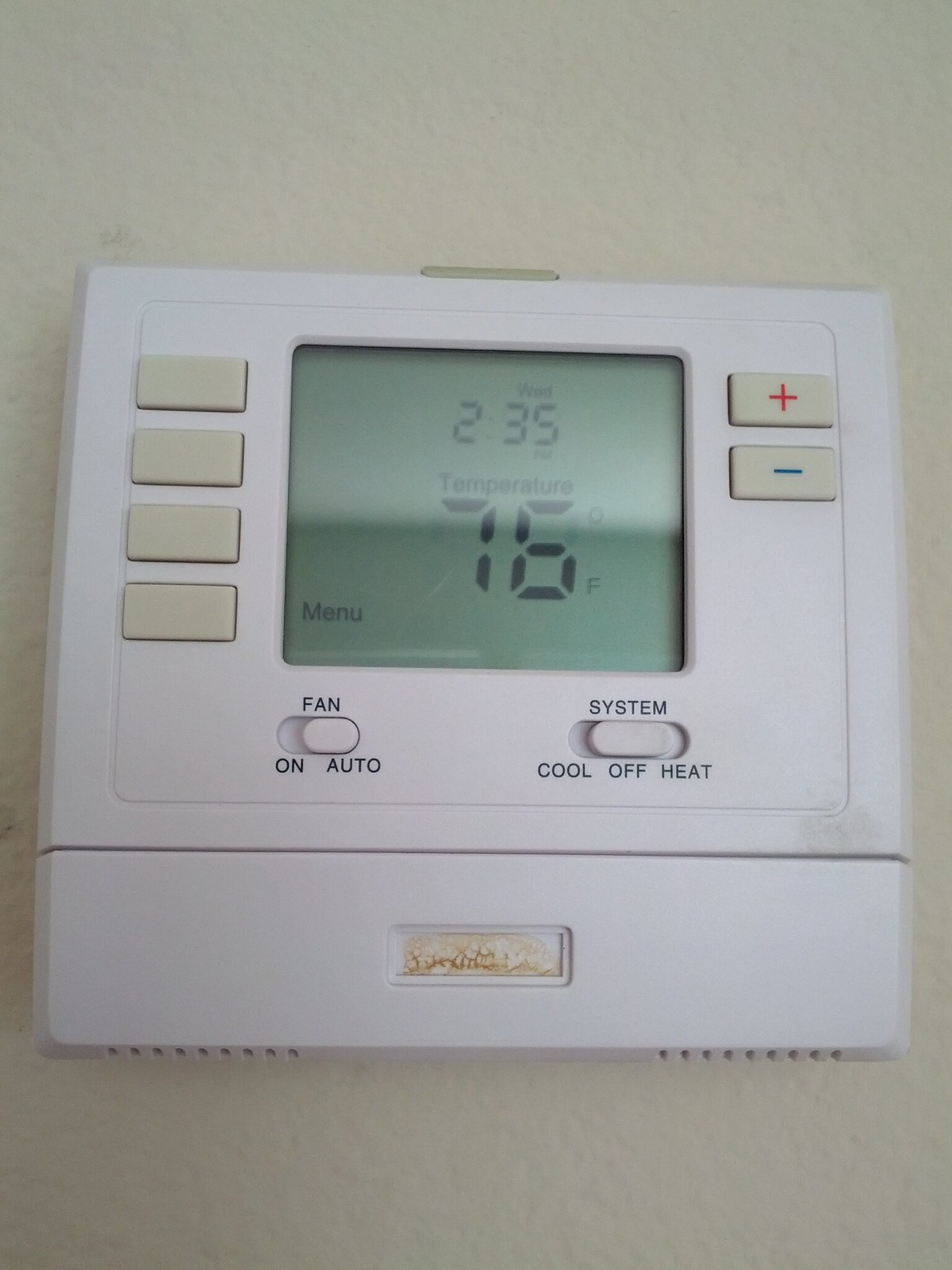This photograph captures a white, slightly off-white plastic thermostat mounted on a gray-green wall. The thermostat features a central panel displaying various pieces of information. To the right of this panel are two buttons: a red plus sign (+) button and a blue minus sign (-) button, likely for adjusting the temperature. Below the central display is a sliding button for controlling the fan settings, allowing the user to switch between 'On' and 'Auto.' On the lower right side, another sliding button marked 'System' enables users to toggle between 'Cool,' 'Off,' and 'Heat' modes. 

The digital display shows a time of 2:35 and a current temperature reading of 76°F. Additionally, near the fourth button on the left side of the unit, the word 'Menu' is displayed, suggesting accessible settings through that control. Beneath the main interface, there appears to be a removable panel, which could potentially be for accessing the thermostat's internal settings or battery compartment.